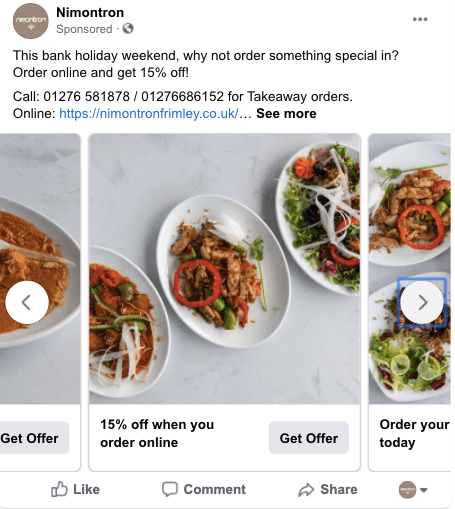This is a detailed caption for the given image:

A vibrant Facebook advertisement from Nimontron (M-I-N-I-M-O-N-T-R-O-N) showcases their latest offering. This sponsored ad promotes a special weekend deal, encouraging customers to order something special for their weekend enjoyment. The ad invites viewers to order online and receive a 15% discount. Detailed contact information is provided for takeaway orders: call 01276 581878 or 01276 686152. Additionally, orders can be placed online via their website: https://nimontronfrimley.co.uk. 

The image features an appetizing arrangement of three colorful plates of food, each meticulously presented on elegant white plates. The dishes include succulent chicken, vibrant peppers, crisp onions, zesty limes, and an assortment of fresh vegetables. A delicate white flower adorns the center plate, adding an extra touch of sophistication. The ad emphasizes the 15% online discount with a prominent call-to-action button to "Get the Offer."